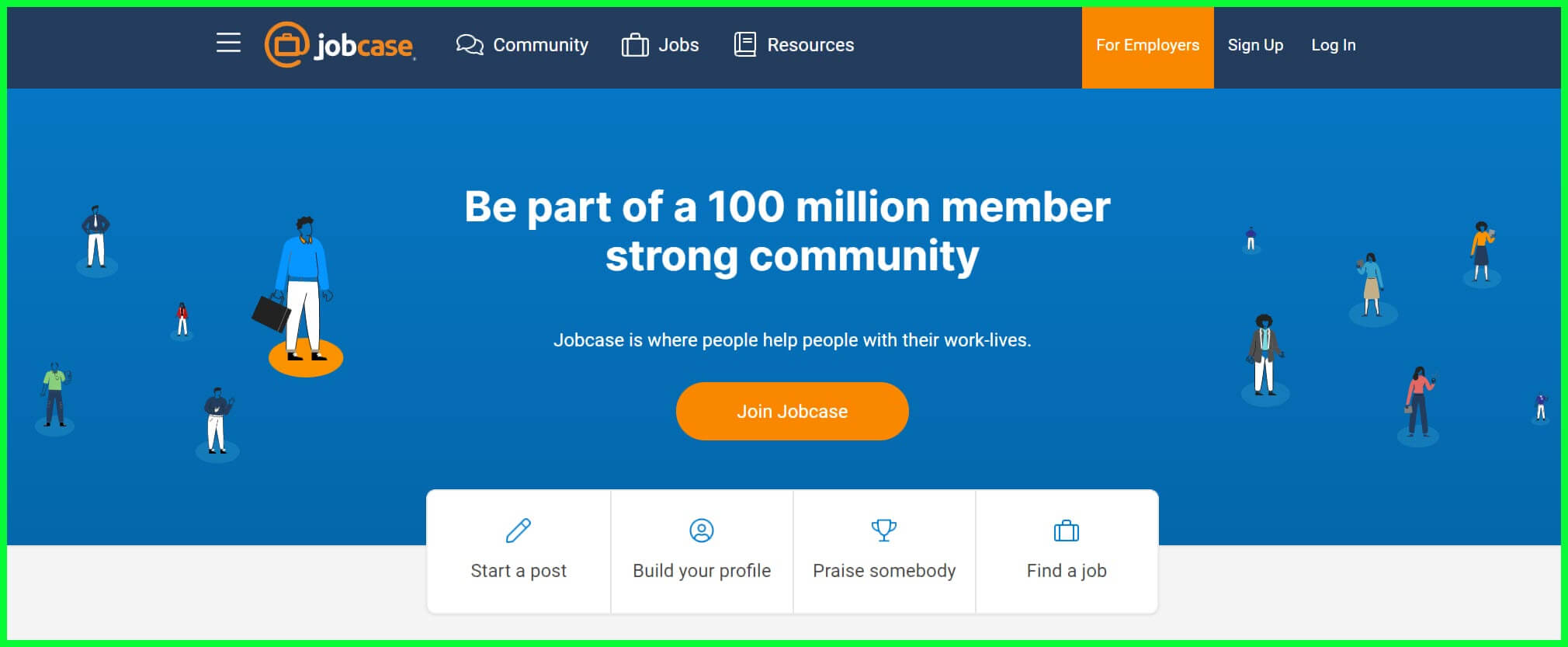This is an image taken from the JobCase website, with "job" in lowercase and white, followed by "case" in orange. The logo is accompanied by an emblem resembling a briefcase, partially encircled by an incomplete ring. The entire image is framed by a green rectangular border.

At the top of the image, "community" is displayed prominently. Alongside in white print are selectable options such as "jobs" and "resources." Also at the top, "for employees" is highlighted in orange, while "sign up" and "log in" appear in regular font.

The main section of the image presents a bold statement: "Be part of a 100 million member-strong community," followed by, "JobCase is where people help people with their work lives." Below this text is an orange button labelled "Join JobCase."

Further down, there are several blue-tinged rectangular buttons with icons. These buttons offer options such as "Start a post," "Build your profile," "Praise somebody," and "Find a job."